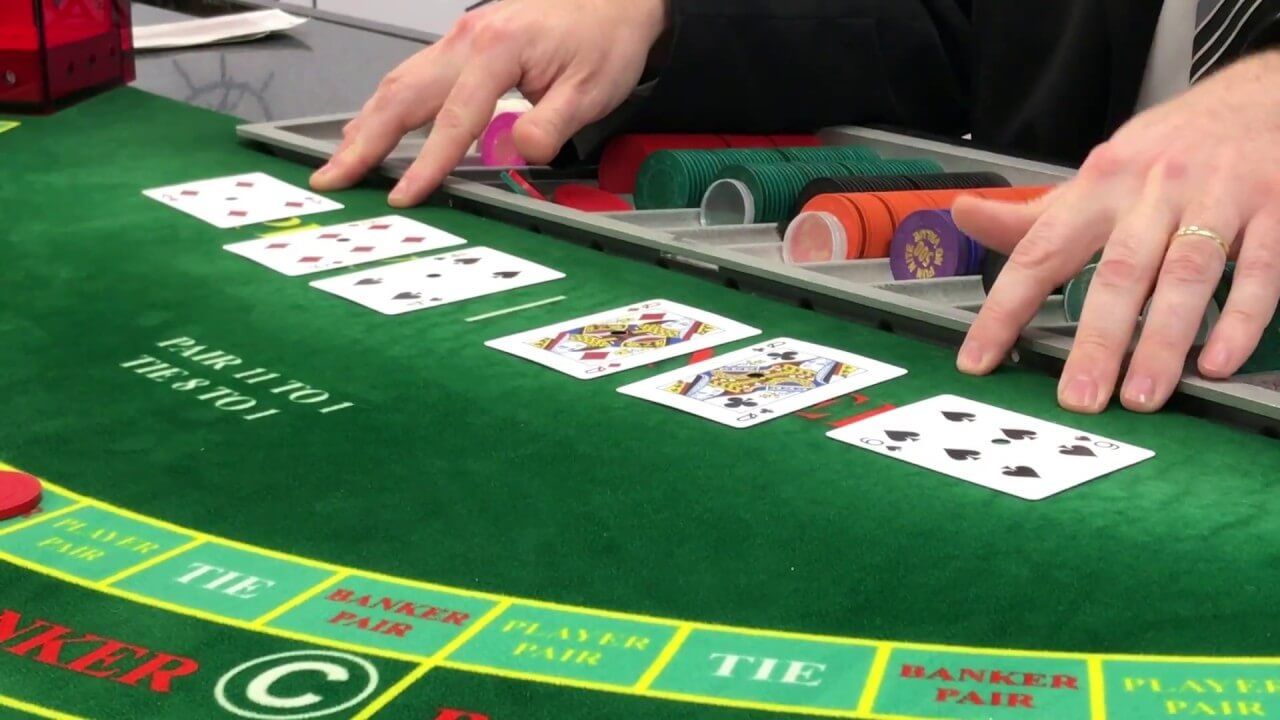The image depicts a detailed setup for a card game on an emerald green tabletop, possibly a variant of blackjack or baccarat. The surface features an ornate layout with distinct sections marked by squares, each labeled with terms such as "Tie," "Banker Pair," and "Player Pair," repeated around the edge. The center of the table bears text like "Pair 11, 10" and "Tie 8 to 10," providing gameplay instructions or payout information. Two groups of cards are arranged on the table: the first group has two cards facing the player and one card pointing to the left, while the second group has two cards aimed at the dealer and one card facing to the right. A player's hands are visible, showcasing a ring on one finger. Additionally, a tray filled with chips is positioned nearby, indicating active gameplay.